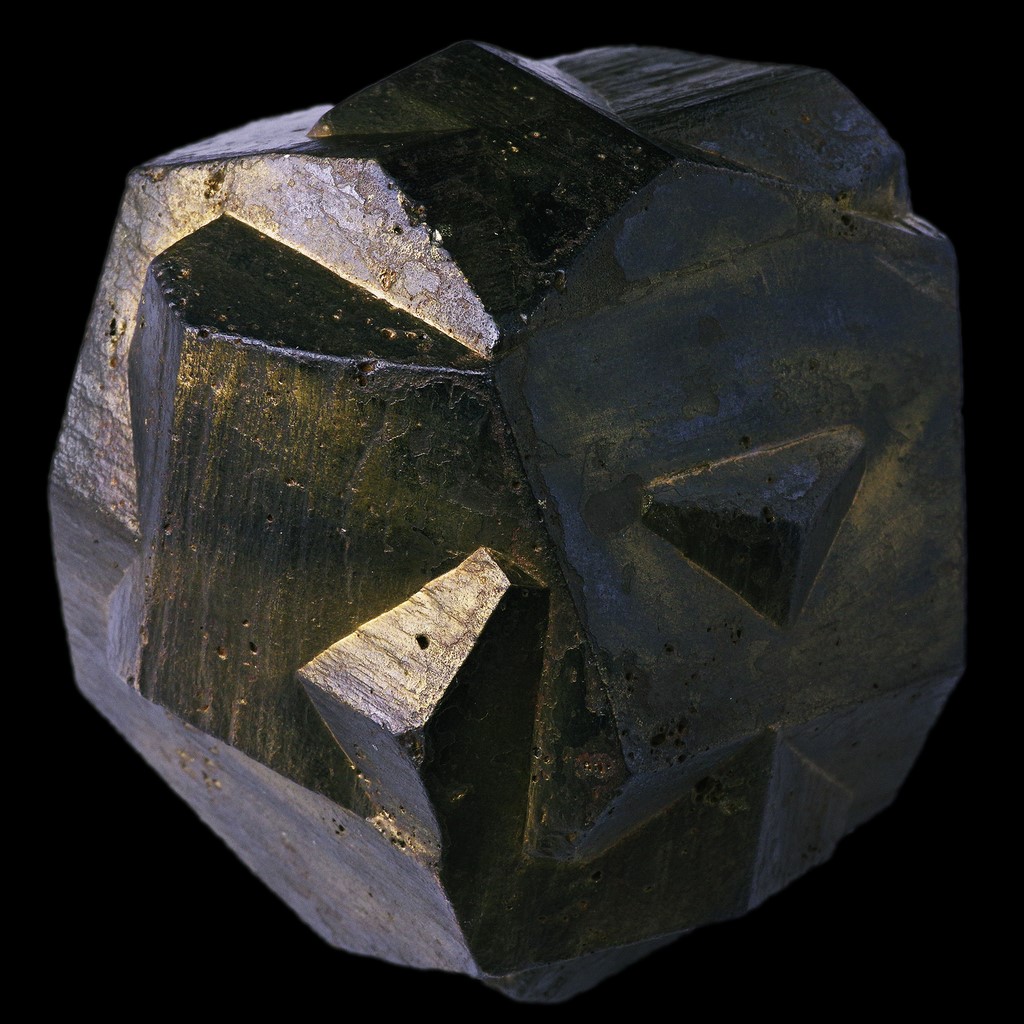This image features a striking and detailed abstract art piece of a rock or metallic mineral specimen, possibly resembling stibnite. The rock exhibits an intriguing convoluted form, intertwining within itself and displaying a variety of distinct angular, triangular, and prism-like features. Predominantly dark black in color, the mineral exudes a captivating golden or even greenish sheen that is highlighted by a light source illuminating one side, while leaving the other side in shadow, accentuating the texture and depth. The rock's surface reveals light pitting and striations of gold and copper. The background is completely black, creating a stark contrast that makes the specimen appear as if floating in deep space. The crystal’s complex, circular structure is punctuated by geometric shapes, including what appears to be a smoothly chiseled pyramid on the right. Every facet and angle of the mineral is clearly defined, making its varied textures and intricate formations strikingly visible.